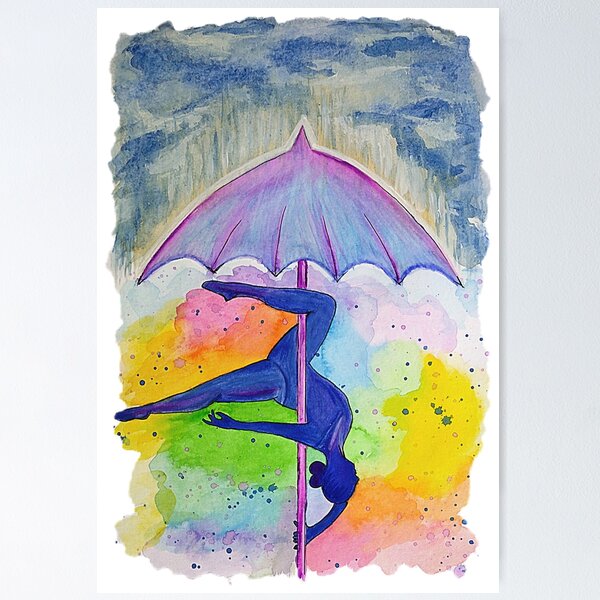The image is a vivid watercolor painting depicting a cloudy, rainy sky. At the center, a girl painted entirely in shades of blue performs acrobatics, gracefully wrapping herself upside-down around the pole of a purplish-pink umbrella. She is dressed in a blue leotard, and her hair is neatly pulled back into a bun. The umbrella, positioned facing upwards, boasts an array of colors including purple, pink, red, yellow, green, and orange, with small dotted details enhancing its whimsical appearance. The background features a dark blue sky, against which the vibrant colors of the umbrella and the acrobat's form stand out sharply. The scene is brought to life with dynamic lines and a sense of movement, emphasizing the dancer's twirling motion and the rainy, cloudy atmosphere surrounding her.